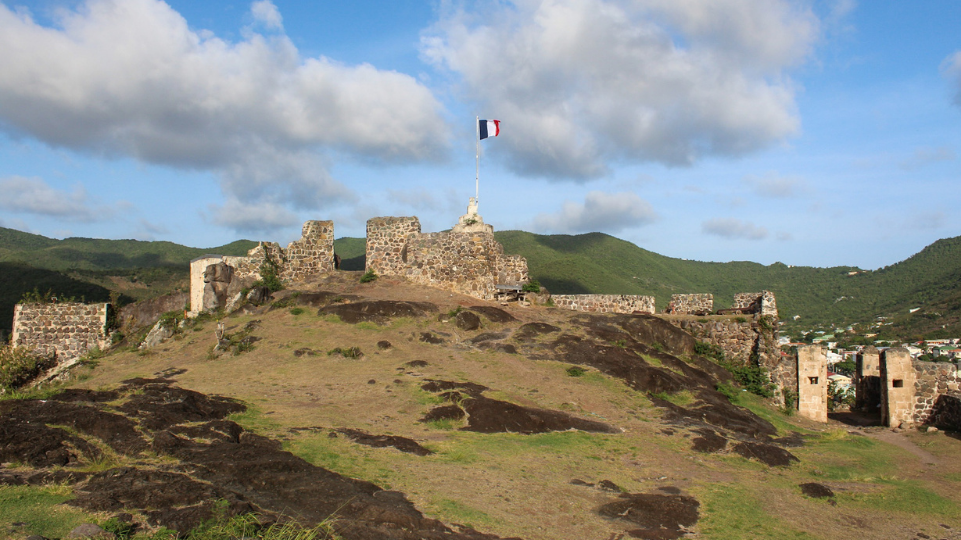The image depicts the remnants of a medieval stone fort set atop a scrabby hill, likely located in France, as suggested by the blue, white, and red vertical stripes of the French flag fluttering atop the highest remnant. The fort, now partially collapsed with broken stone walls, features an entryway on its right side, marked by two standing columns. The foreground consists of patches of barren dirt interspersed with dead grass, lending a rough texture to the hill. In stark contrast, the background reveals a serene landscape of shallow green hills under a mostly clear blue sky with a few puffy white clouds, suggesting a beautiful summer day. The distant settlement peeks through the greenery, framing the historic fortifications against a picturesque natural backdrop.